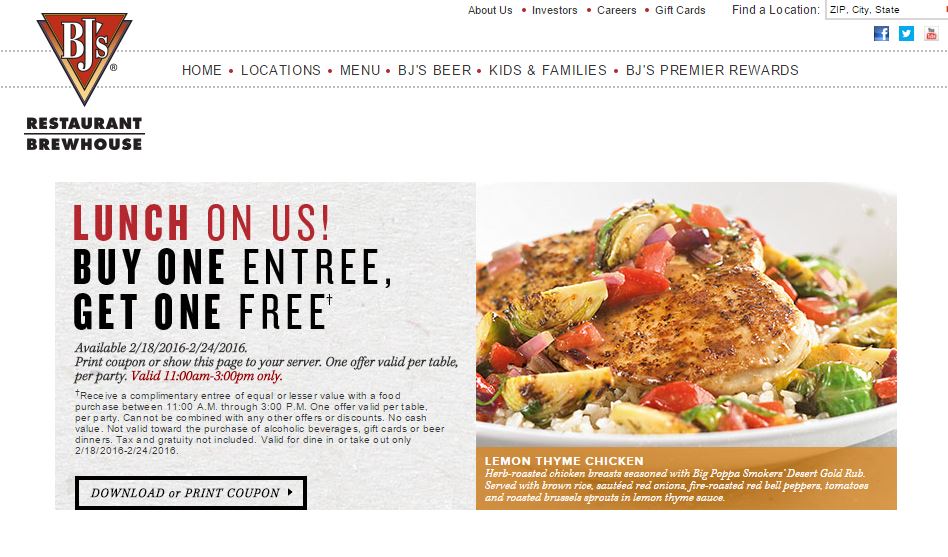The top-left corner of the page features BJ's Restaurant and Brewhouse logo, consisting of a red triangle overlaying a yellow triangle with white "BJ's" text on top. Below the logo, "Restaurant" is written in black font, followed by a line, and then "Brewhouse."

A navigation bar extends from beneath BJ's logo, listing the following options: Home, Locations, Menu, BJ Beers, Kids and Family, and BJ's Premier Rewards. Above this in the top-right corner, there are additional links: About Us, Investors, Careers, Gift Cards, and Find Locations. Next to these links is a search field labeled, "Zip, City, State."

Between the two navigation rows are social media icons for Facebook, Twitter, and an unidentified third platform.

The web page has a white background. On the lower left, there's a promotional offer stating, "Lunch on Us: Buy one entree, get one free, available from 2-18-2016 through 2-24-2016." Instructions specify to print the coupon or show the page to the server, with the valid times (11 a.m. to 3 p.m.) highlighted in red. The terms detail that one offer is valid per table or party, providing a complimentary entree of equal or lesser value. It cannot be combined with any other offer or discount, holds no cash value, and is not applicable towards alcoholic beverages, gift cards, or beer dinners. The offer is only valid for dine-in or table takeout and excludes tax and gratuity. The exact dates and additional instructions regarding downloading or printing the coupon are reiterated at the end.